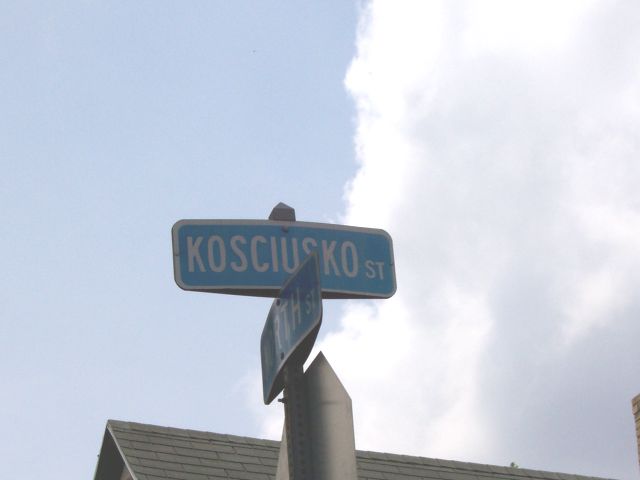The image showcases two intersecting street signs set at right angles against a picturesque outdoor backdrop. Dominating the center, the upper sign clearly spells out "Kosciuszko Street," while the lower sign, slightly angled and more challenging to decipher, ends with "RTH Street," likely indicating "4th Street." The background features a serene scene, with a clear blue sky occupying the left-hand portion and fluffy white clouds adorning the right, capturing the essence of a bright daytime sky. At the bottom of the frame, the gray slate roof of a nearby house adds a touch of domestic life to the composition.